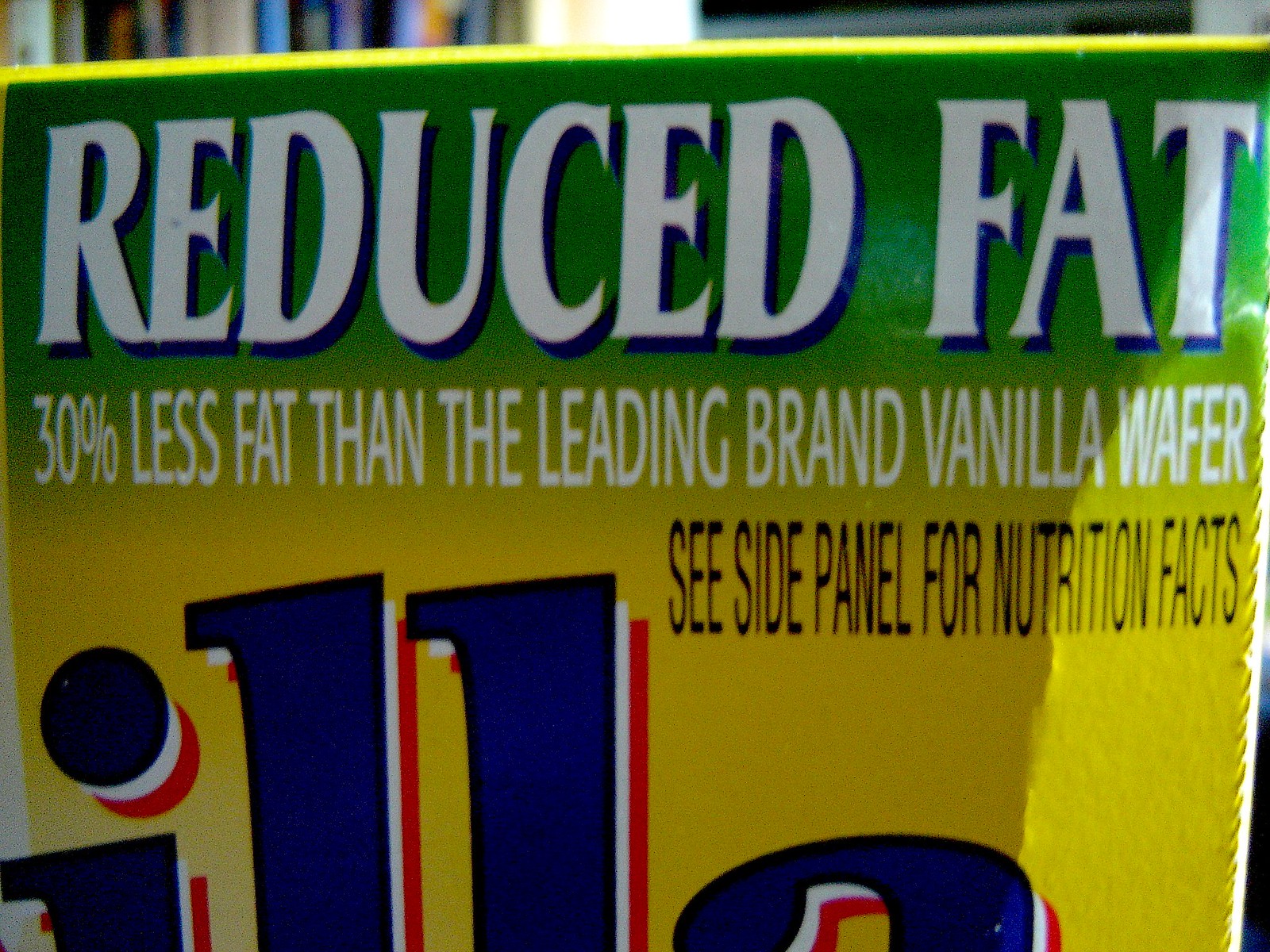This image is a close-up photograph of a colorful label or sign, likely designed for a food product box. The label features a top border outlined in bright yellow, which fades into a green background. At the top, large white letters spell out "Reduced Fat," with a 3D effect created by blue shadowing. Below, the label states "30% less fat than the leading brand Vanilla Wafers." In the lower part of the image, text in bold black letters advises, "See side panel for nutrition facts." Further down, partially visible letters "I-L-L-A" are styled in white with blue borders and a red 3D effect, although they are cut off. The background includes various brightly colored objects resembling books or folders, adding a vibrant, busy atmosphere to the label's surroundings.